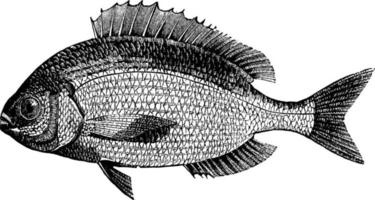This detailed black-and-white ink drawing illustrates a fish facing left, meticulously capturing a classical, hand-drawn style. Every scale is rendered with precision, providing a textured, lifelike quality to the fish's side profile. The fish features a prominent spiky fin running along its back, accompanied by a similarly spiky ventral fin near its lower rear. Distinctively, the fish's darker face and V-shaped tail contrast with the lighter shading of its midsection. The top fin, while somewhat lighter than the fish's upper body, still stands out against its silvery belly. Both pectoral fins show a gradient, light at the top and darkening toward their tips. This illustration's intricate detailing, from the dark eye to the delicate mouth, showcases a harmonious blend of light and shadow, making the composition striking against a white background.